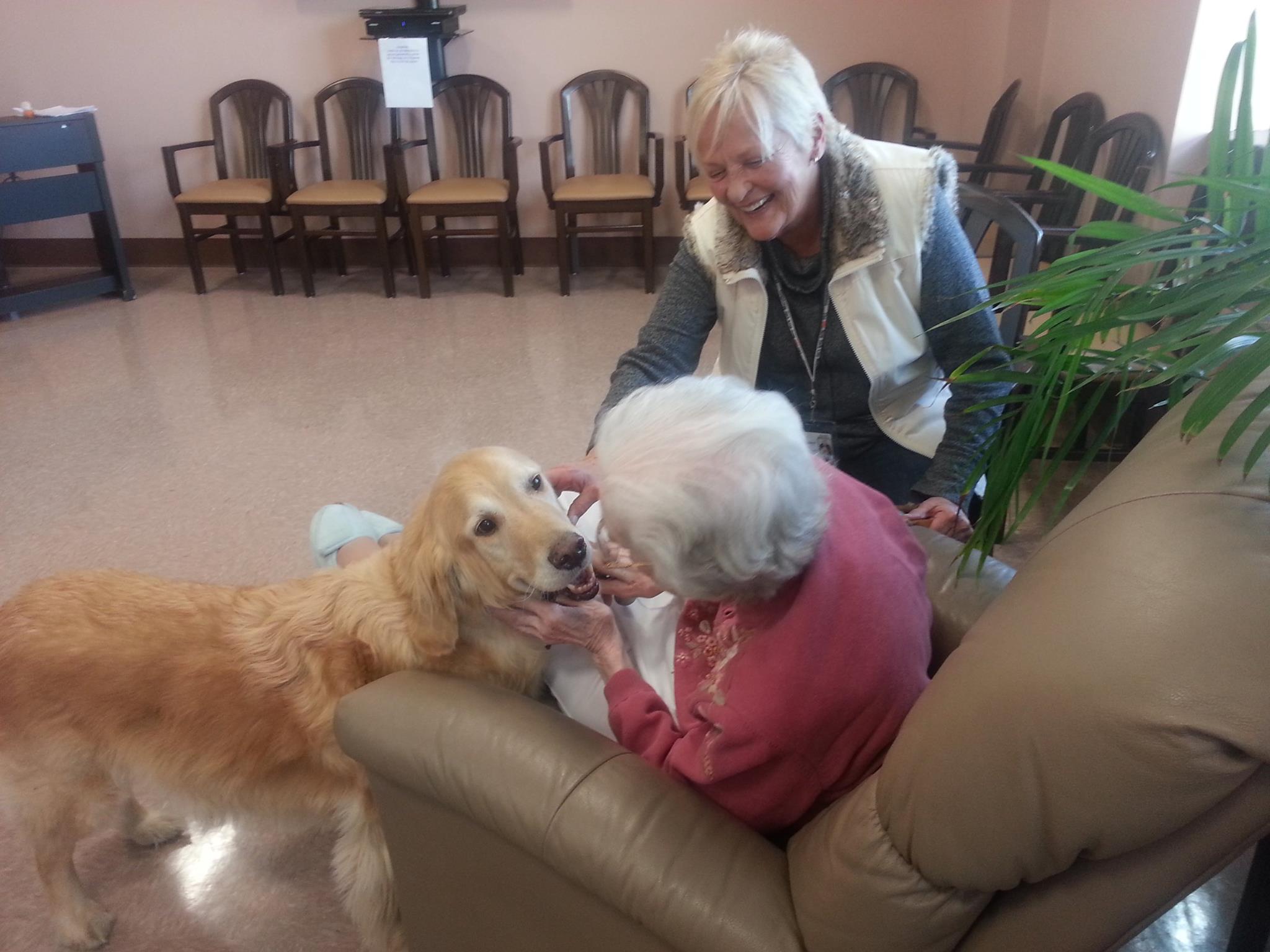In a cozy, well-lit room, two women, seemingly in a nursing home, share a tender moment with a golden retriever. The elderly woman sitting on a brown leather couch, dressed in a pink sweater and white trousers, affectionately pets the furry, golden-brown dog, which gazes back at her with a friendly expression. Beside her, another woman with short white hair, clad in a white sleeveless coat over a blue long-sleeved shirt and wearing a long necklace, stands laughing and admiring the scene. The room’s decor includes a potted plant with green blades on the right side, brown tile or marble floors, a row of brown chairs lining the wall in the background, and a table in the top left corner. The photograph captures a heartwarming moment of joy and companionship among the women and their loyal canine friend.